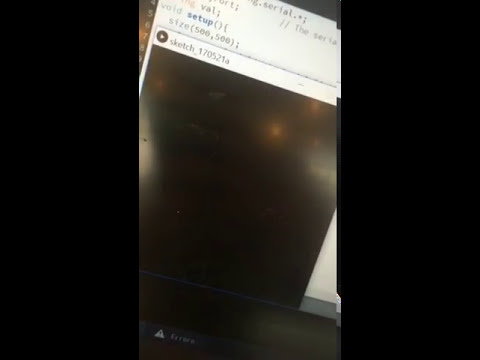The image features a skewed, shiny rectangular screen, most likely a computer display, with a distinctive black background and white text at the top. The text includes coding elements such as "Serial," "Val," "Void Setup," "Size(500, 500)," and "Sketch_170521A." Near the upper left corner, partially obscured, are the numbers "5678" and part of a "9." The screen displays a blank, black area beneath the white text. At the very bottom, there's an error indicator, shown as a triangle with an exclamation mark and the word "Error" next to it. The screen is centrally placed within the image, flanked by wide, black borders on the left and right sides, with no borders at the top and bottom. The overall setting suggests a technological environment, possibly depicting an error in a coding or programming interface.